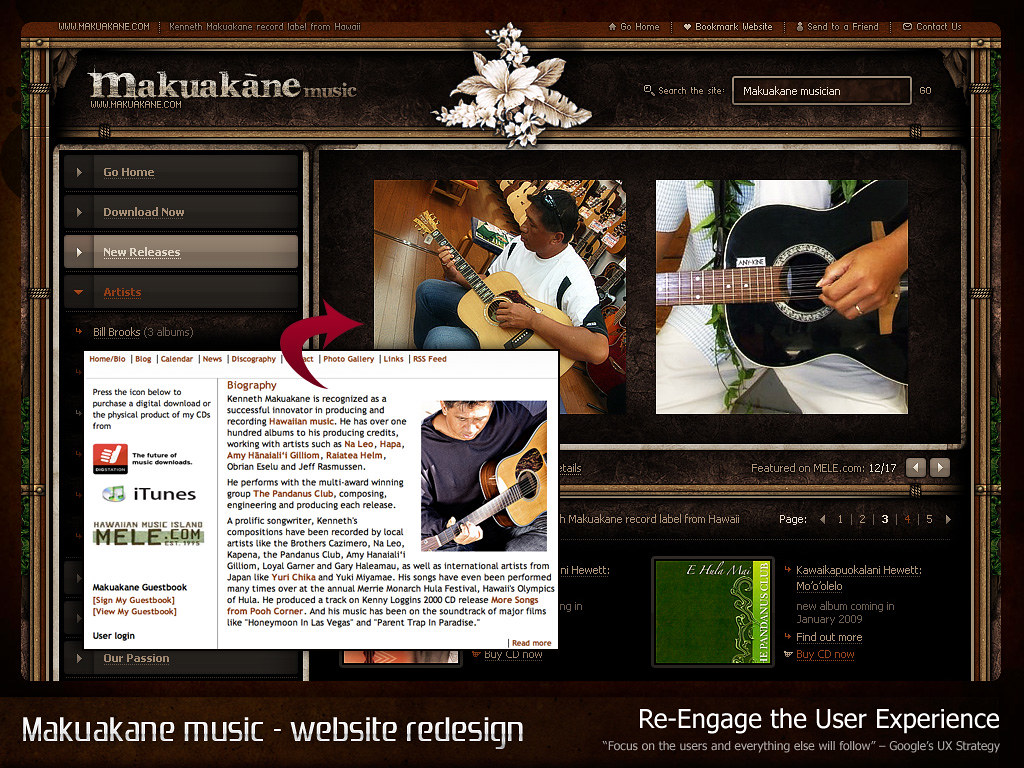The image appears to be a detailed screenshot of the Makuakane Music website, showcasing its unique and somewhat busy interface. At the top, the website header displays "Makuakane Music" in whitish letters, with several navigation options including 'Go Home,' 'Bookmark Website,' 'Send to a Friend,' 'Contact Us,' 'Download Now,' and 'New Releases.' The background theme is predominantly brown, adorned with flower decorations, notably a white bouquet in the center.

Featured prominently are various images related to Hawaiian music. There's a picture of a light-skinned man in a purple long-sleeve sweatshirt playing a tan guitar with a black and orangish pickguard. Another image shows a dark-skinned man playing a similarly designed guitar, positioned in what looks like a guitar shop with a dark wood floor and guitars displayed on the wall behind him. Additionally, there's a close-up of a woman's hand, identified by a manicured fingernail and a diamond ring, playing a black-faced guitar.

A red arrow points to a section with an article or biography about Kenneth Makuakane. It acknowledges him as a successful innovator in producing and recording Hawaiian music. Various clickable elements are scattered throughout the interface for purchasing albums, songs, and possibly accessing music via iTunes and MELE.com, promising an engaging user experience on this redesigned website.